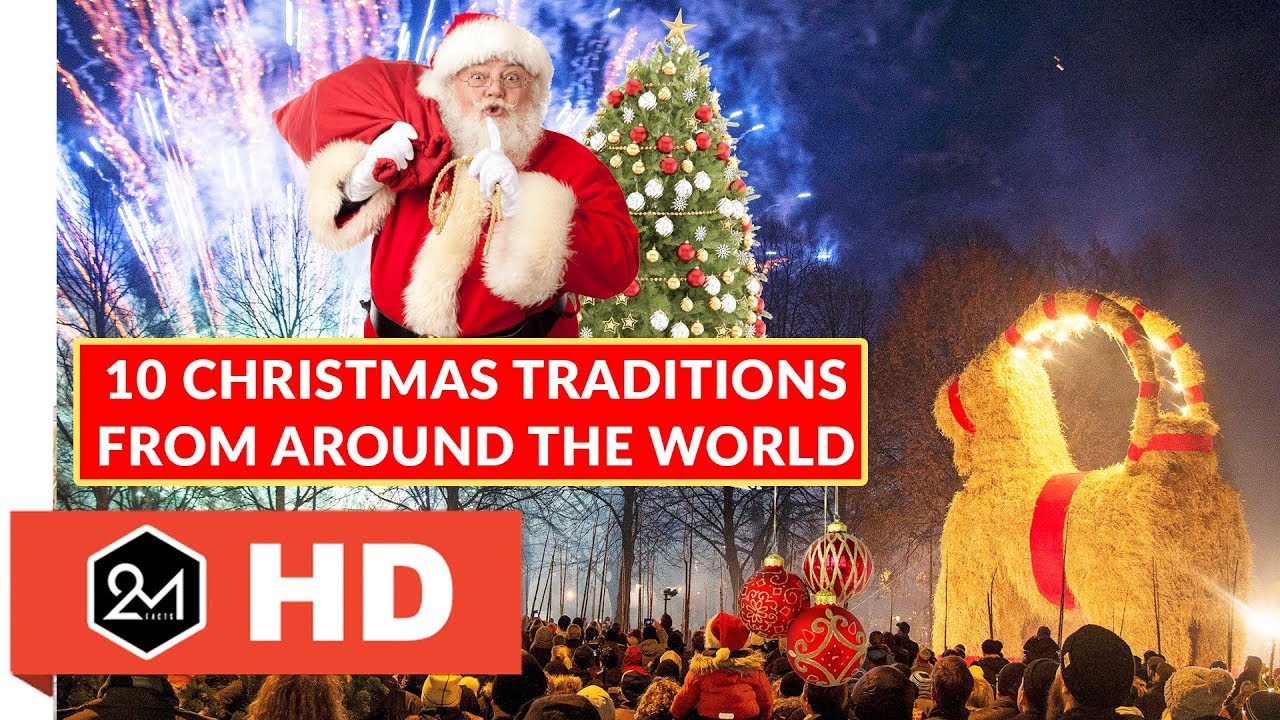The image features a vibrant and festive Christmas poster with a central theme of "10 Christmas Traditions from Around the World." The background is predominantly red, emphasizing the holiday spirit. Santa Claus, dressed in his classic bright red uniform adorned with white fur trim and white gloves, occupies the upper left quadrant. He carries a sack over his shoulder and gestures with a finger to his lips, suggesting silence. Behind him, a decorated Christmas tree with red and white ornaments and a star on top stands in contrast to the blue firework-lit sky.

In the foreground, a diverse crowd of people, some wearing Christmas attire, gather in what appears to be a park. They are all facing away towards a spectacular firework display, adding a sense of celebration. To the right, there is an imposing straw sculpture resembling an animal, possibly a goat or horse, with distinctive thick legs, red accents, and curved horns.

The prominent red banner at the bottom of the poster reads “10 Christmas Traditions from Around the World” in white letters. An additional red banner below it includes some markings and an indistinct logo, possibly reading "2MHD." Trees without leaves frame the scene, completing this dynamic and joyous depiction of international festive traditions.